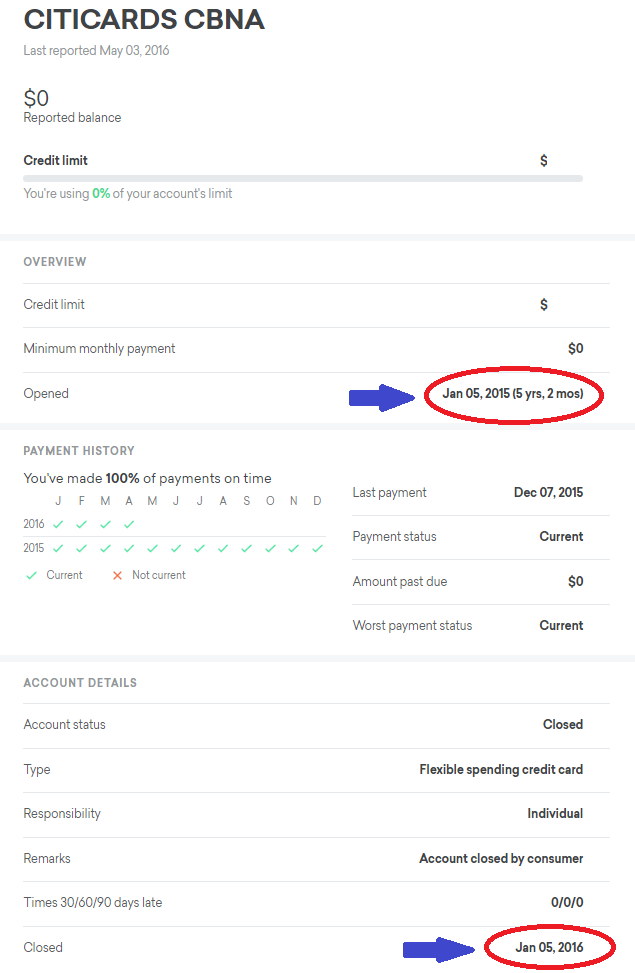This detailed image captures a screenshot of a CityCard's CBNA account summary. The latest update on the account was on May 3rd, with the reported balance being zero, and the credit limit utilization showing zero percent. The overview section confirms that the credit limit and minimum monthly payment are both zero.

A significant portion of the image focuses on the date the account was opened, January 5th, 2015, highlighted with a prominent red circle and a blue arrow. The duration, noted as five years and two months, is visible nearby.

The payment history section indicates the last payment was made on December 7th, 2015, with the payment status marked as current and zero past due amount. The record shows the worst payment status as current as well.

Further account details reveal the account status is closed, cited as a flexible spending credit card under individual responsibility. The remarks state the account was closed by the consumer. The account faced no late payments—shown as 30, 60, and 90 days late all marked as zero. Finally, another date, January 6th, 2016, representing when the account was closed, is also emphasized with a red circle and a blue arrow.